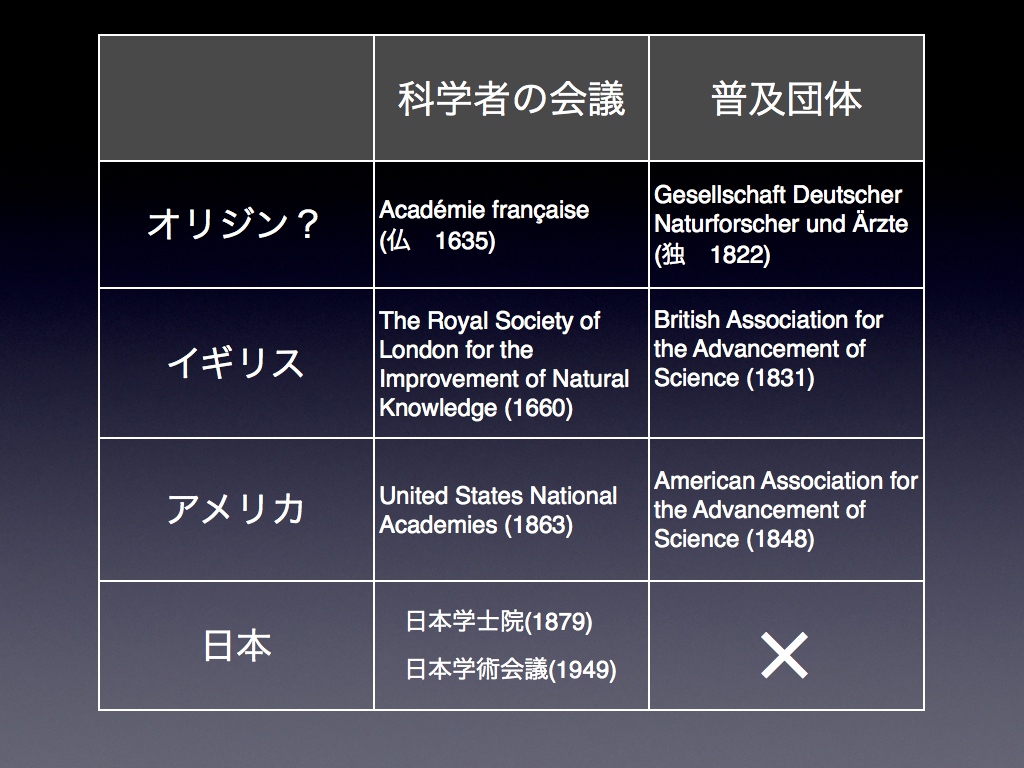This detailed digital image appears to be a PowerPoint-style slide with a dark navy blue background and a grid comprising three columns and five rows. The topmost row features three gray boxes, the first of which is blank, while the second and third contain text in an East Asian language, likely Japanese. The subsequent rows include a mix of textual elements in various languages.

The first column displays text written in the same East Asian language within each of the bottom four boxes. In the second column, the second row contains text in English: "Académie Française (1635)." The third row reads: "The Royal Society of London for the Improvement of Natural Knowledge (1660)." The fourth row states: "United States National Academies (1863)." The final row includes two lines of text in an East Asian language, labeled with the years "1879" and "1949."

The third column’s second row features German text: "Gesellschaft Deutscher Naturforscher und Ärzte (1822)." The third row reads in English: "British Association for the Advancement of Science (1831)." The fourth row states: "American Association for the Advancement of Science (1848)." The final box in this column contains a simple X mark.

This comprehensive image shows an organized chart detailing various academies and scientific societies from around the world, set against a dark blue background for clear visual contrast.